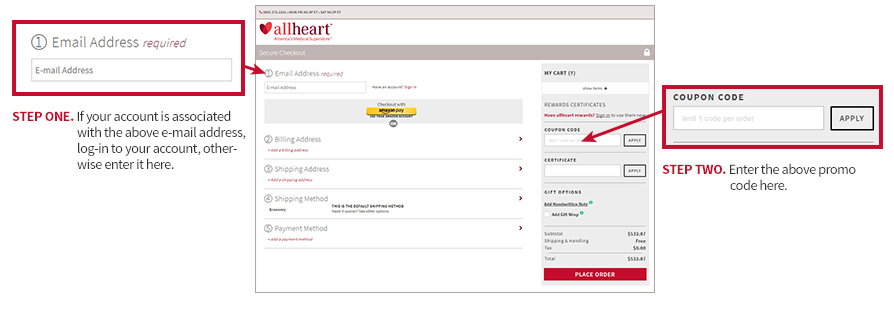"On this page from the AllHeart® website, America's medical supplies provider, we observe a user login and discount redemption interface. To the left, there is a section requiring an email address, featuring a bar designed for input. Step one prompts users to log in with the associated email address or enter a new one if it hasn’t been previously registered. The name 'AllHeart, America's medical...' is partially visible, but some text is blurred. To the right, there is a field labeled 'Step two' instructing users to input a promo code above the 'Coupon Code' label. The drawing attention to the vibrant coupons colored in red, grey, and yellow contrasts against an otherwise predominantly white background."